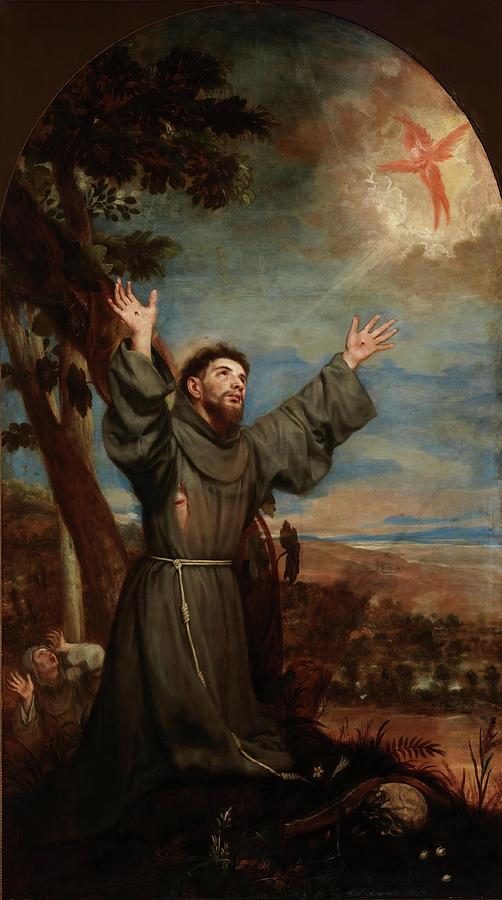This intricately detailed oil painting from possibly the 16th or 17th century, features a stirring religious scene. At the center, a bearded monk in a dark greenish-gray or black robe, secured with a rope belt, kneels with his hands outstretched upward. Bloody stigmata are evident on his palms, and his tear in the robe reveals a cut beneath, an imagery reminiscent of Christ's crucifixion wounds. His gaze is directed to the sky, where he appears to be praying to an angelic figure amidst the clouds, a red cherub or baby with wings. Light emanates from the angel, illuminating the devout monk's head and upper body. Below and to the left of the monk, another figure stands with hands near their ears, seemingly in shock at the heavenly vision. The backdrop is dark, punctuated by a partial moon, sparse clouds, and a few brushed trees, adding to the somber yet mystical atmosphere. The painting, arched at the top, might adorn a wall and contains a rich palette of green, brown, blue, white, pinkish-red, and black hues, but no text or numbers, focusing solely on this profound religious moment.